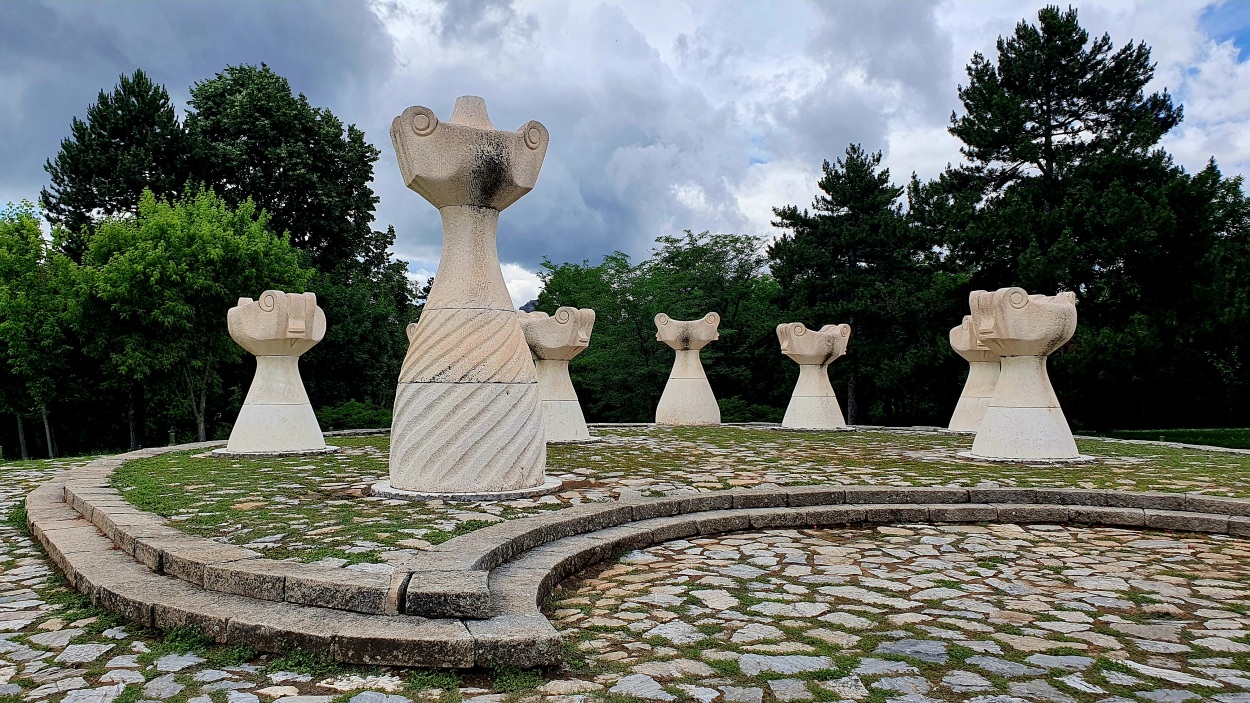The professionally-taken photograph captures an outdoor setting in what appears to be a public garden or historical mansion grounds with a semi-cloudy sky and patches of blue. The scene is composed of a picturesque, two-tiered platform made of cobblestones interspersed with grassy patches and moss. Dominating the foreground are at least seven stone sculptures, resembling oversized chess pieces or ornate vases, each featuring a tapered base culminating in a head-like top with simplistic facial features, such as circular eyes. The sculptures, approximately 10 feet tall and shaded sandy off-white with black and gray accents, sit prominently on a grassy, elevated stone platform akin to granite. In the background, a dense tree line of tall, proud evergreens frames the scene, completing the tranquil, verdant park-like atmosphere. The absence of people, animals, or signage contributes to the serene and undisturbed nature of the image.